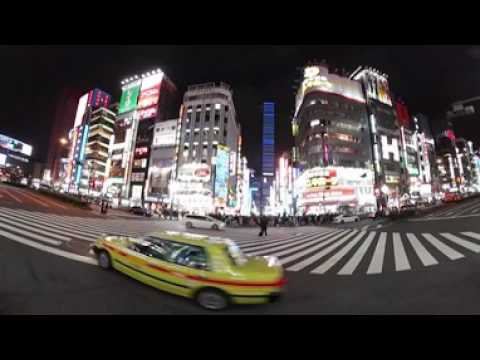The image depicts a bustling, nighttime city scene with a panoramic, slightly distorted view. Prominently featured in the foreground is a yellow taxi with red and green stripes, moving toward a crosswalk marked by white stripes on the road. Pedestrians walk along the crosswalk, creating a sense of movement and activity. A white vehicle appears to be approaching a person, though the distortion exaggerates this interaction. The background showcases a vibrant cityscape with numerous tall buildings illuminated in various colors—reds, greens, blues, and yellows—against a pitch-black sky, implying it is nighttime. Some buildings display neon signs, possibly containing Asian characters, and one prominent building features a bright, glowing 'H,' indicating a hospital. The street is filled with more traffic, and people in dark clothing are visible. Despite the blur and distortion, the photograph captures the lively essence of a major city, possibly in Asia, lit up by electrifying lights and bustling with nighttime activity.